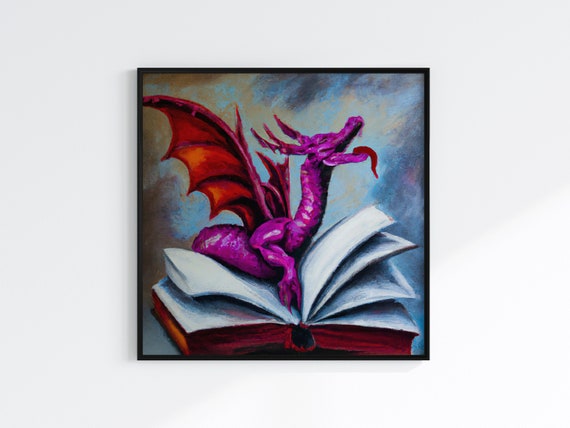The image showcases a detailed painting or drawing in a thin black frame, hung on a blank white wall. At the center of the artwork is a vibrant pinkish-purple dragon, adorned with red wings and horns. The dragon is depicted with its mouth open, revealing a long red tongue. It is nestled between the open pages of a book with a red cover, appearing to hold the book open. The composition features a dynamic mauve, blue, and orange background with splashes of gray and white, enhancing the fantastical elements. The dragon gazes upward towards the top right corner of the frame, capturing an air of whimsy and magic.